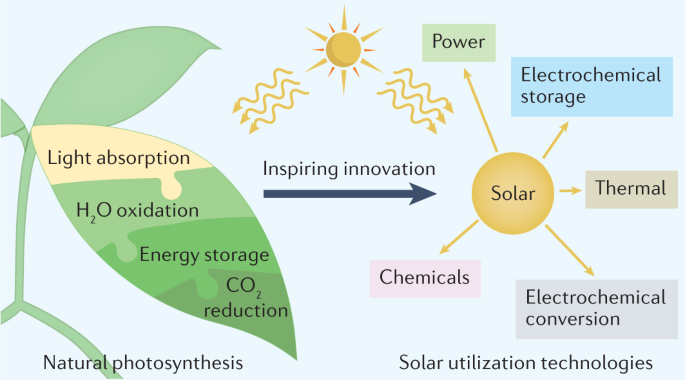This detailed infographic illustrates the process of photosynthesis and its technological applications. The left side depicts natural photosynthesis in a plant, showcasing key components: light absorption, H2O oxidation, energy storage, and CO2 reduction. A large yellow sun at the top center emits light rays—depicted as yellow squiggly lines—towards both the plant and a central circle labeled "solar." An arrow labeled "inspiring innovation" connects the plant to the solar circle. From the solar circle, five arrows extend to various solar utilization technologies: a green box indicating power, a blue box for electrochemical storage, a beige box for thermal energy, a gray box for electrochemical conversion, and a pink box for chemicals. The background features a light blue color reminiscent of a sky or clouds, underscoring the thematic connection to natural processes. The bottom left is marked with "natural photosynthesis" while the bottom right is labeled "solar utilization technologies," tying together the natural and technological aspects of light-based energy transformation.